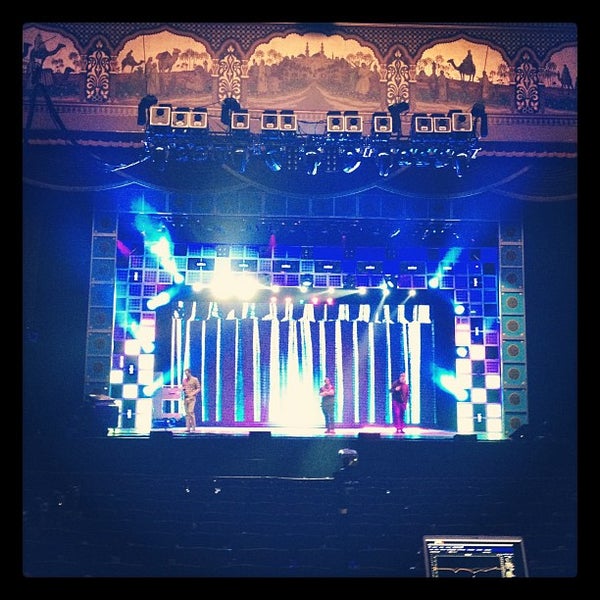This detailed image captures a brightly lit stage set in a theater. Vibrant blue, green, and pink lights illuminate the stage, creating a dramatic contrast against the dark foreground, which appears to contain seating. In the bottom right corner, a computer screen is visible, possibly controlling the stage lights or sound system. On the stage, three people are positioned: one on the left, one in the middle, and one on the right, with the leftmost individual donning a tan outfit. The backdrop features a black and white curtain surrounded by small squares that seem to both emit and reflect the colorful lights. Above the stage hangs a set of twelve speakers, providing robust sound coverage. Crowning the scene is an intricate mural with tannish hues that depicts a scenic Middle Eastern tableau, complete with camels, men, and trees, adding an ornate and exotic ambiance to the performance venue.